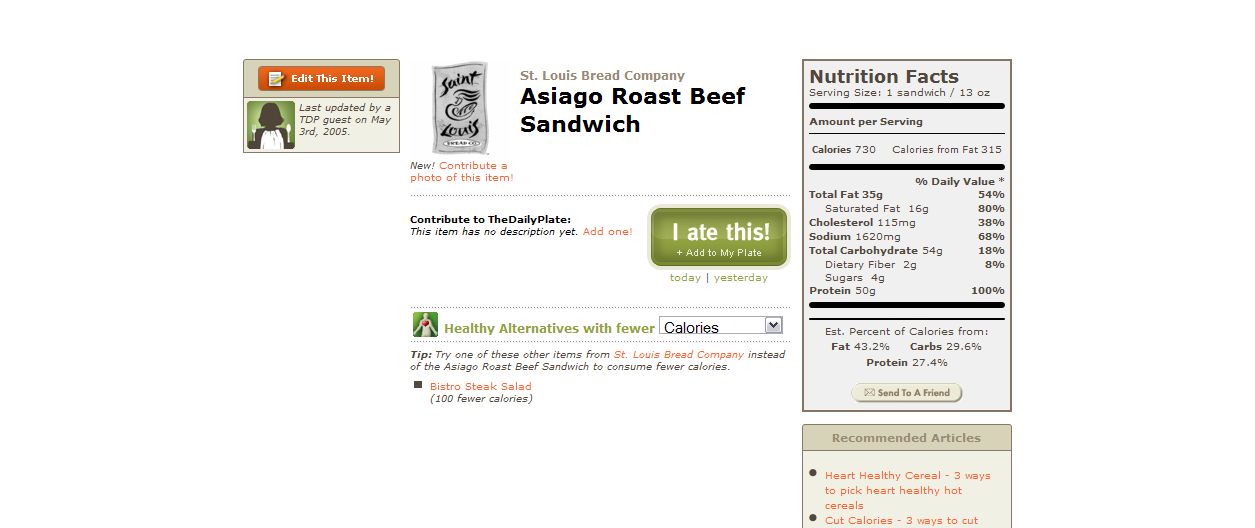This image is a screenshot from the Daily Plate app, a popular calorie and food tracker. It displays the nutritional information for the St. Louis Bread Company Asiago Roast Beef Sandwich. The image shows a green "I Ate This" button, allowing users to easily add the item to their daily food log. Detailed nutrition facts are prominently featured, including total fat, cholesterol, sodium, total carbohydrates, dietary fiber, sugars, and protein content. The app also suggests related articles for further reading and offers a pull-down menu for selecting healthier alternatives with fewer calories.